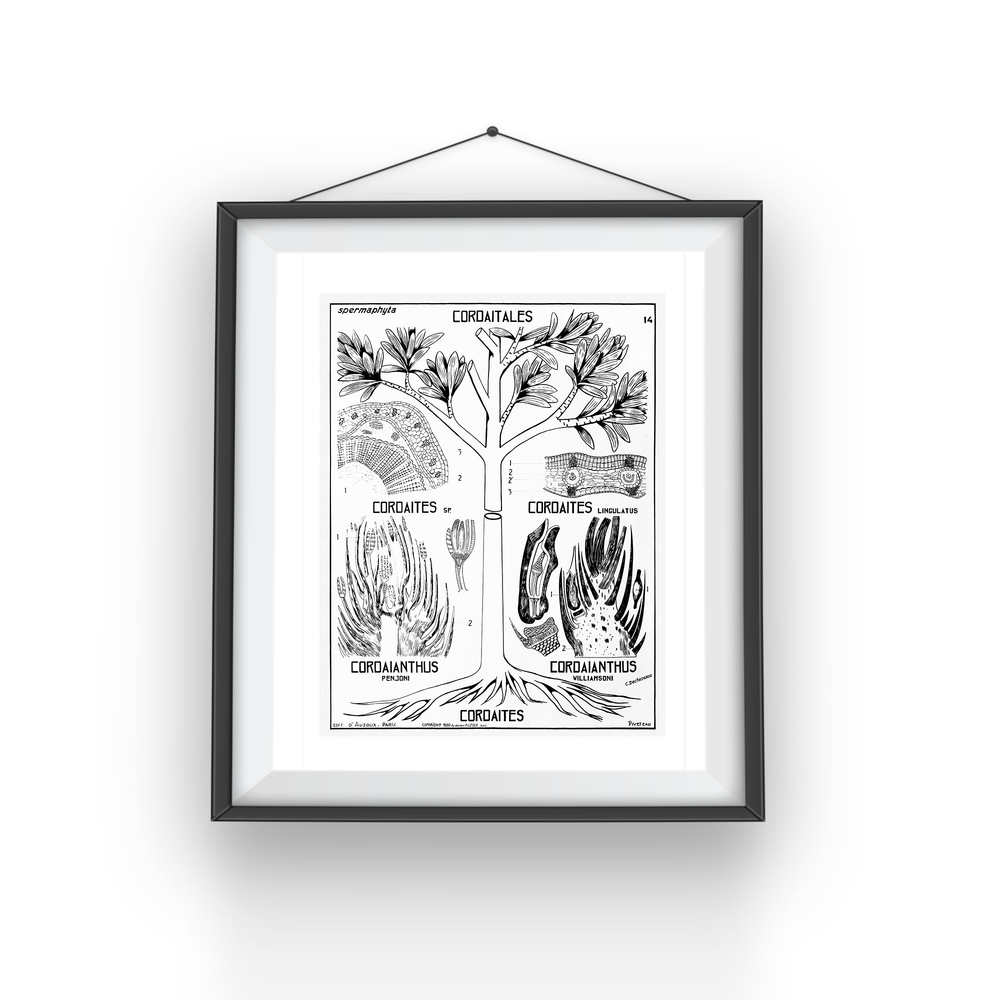Hanging on a wall is a framed botanical illustration, meticulously done in black line art. The black frame encases a detailed sketch of a tree, its branches, leaves, and roots intricately depicted. The artwork is divided into various sections, each showcasing different parts of the tree, including detailed internal structures of leaves and possibly the wood or vines. At the bottom, there's a series of individual schematics providing close-up views of the botanical elements. The Latin term "cordatalis" is repeated multiple times across the illustration, though its exact meaning is unclear. Additionally, the term "spermaphyta" is inscribed at the top. The artwork also appears to be numbered and signed, emphasizing its crafted nature. The overall design is both scientific and aesthetically refined, indicating a blend of artistic precision and botanical knowledge.